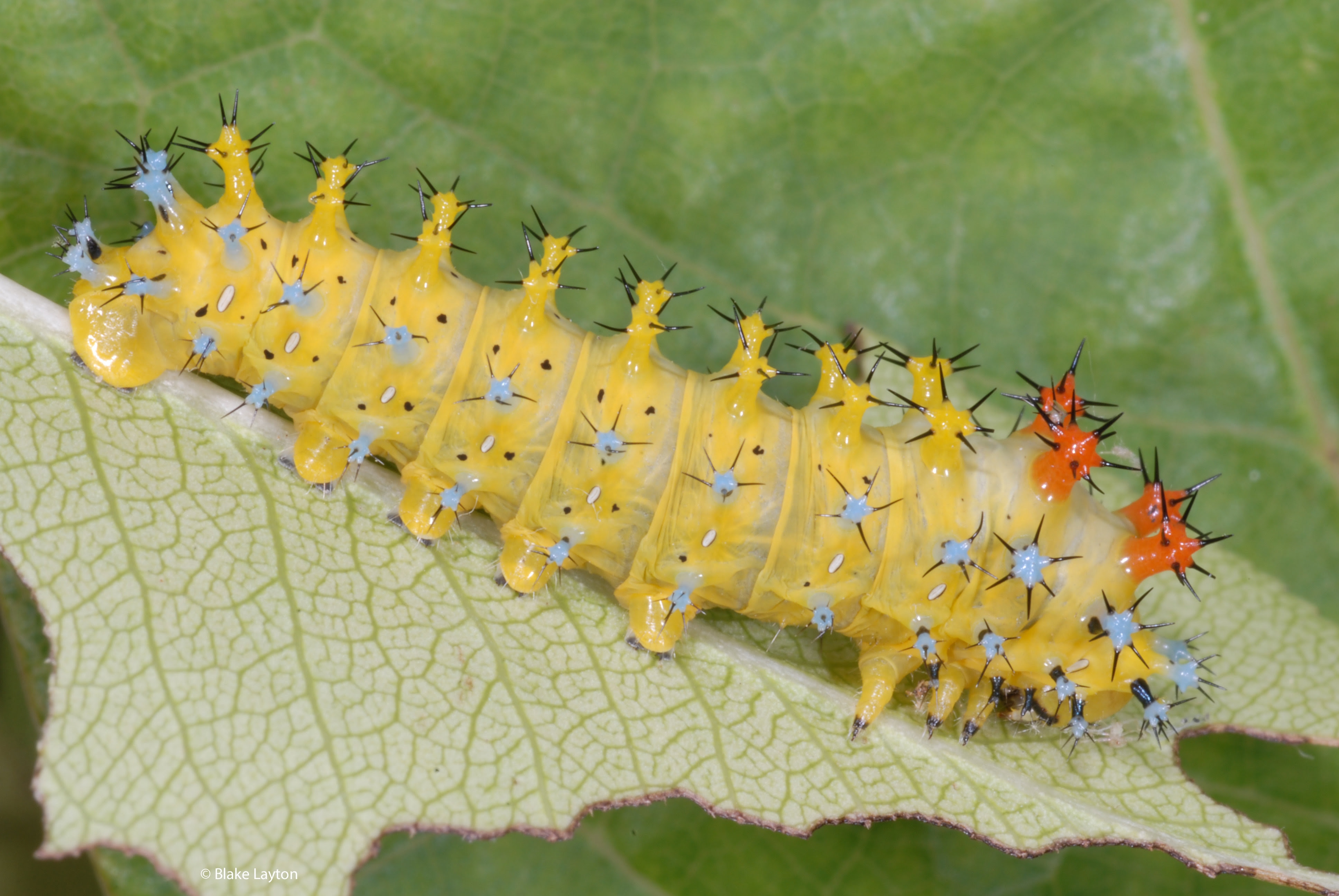In this vivid photograph taken at Lake Layton, a striking yellow caterpillar is prominently displayed on a green leaf. The caterpillar, seemingly happy and possibly munching on the leaf, is adorned with a mesmerizing array of spikes. Most of these spikes are yellow, but some are tinged with vibrant blue and fiery orange hues, each tipped with sharp black points. The intricate pattern of the caterpillar's body includes bulbous protrusions at one end that are particularly colorful with orange and blue accents, giving the illusion of eyes and creating a captivating visual effect. While the exact orientation of the caterpillar isn’t clear, its vivid colors contrast starkly against the lush green leaf, making the creature stand out dramatically. The composition of the image, with its detailed focus and natural setting, perfectly captures the essence of this extraordinary insect in its natural habitat.